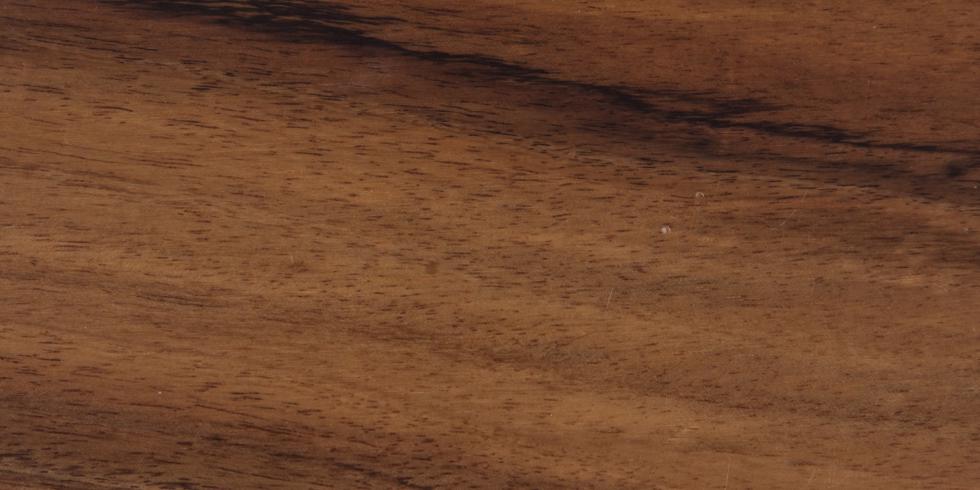The image displays a highly detailed close-up of a wooden plank, filled with intricate wood grain patterns that extend horizontally across the entire frame. Its overall color is a rich brown, with a matte finish that lacks any shine, suggesting a natural, untreated surface. A prominent darker streak runs from left to right, adding a striking contrast to the predominantly tan and brown hues. Flecks and spots are scattered throughout, adding texture and depth, with darker areas towards the top and bottom left corner. The impression of waves of lighter color towards the center creates a dynamic visual effect. The meticulous detail suggests a very magnified or closely focused photograph, capturing the familiar textures and markings characteristic of wood.